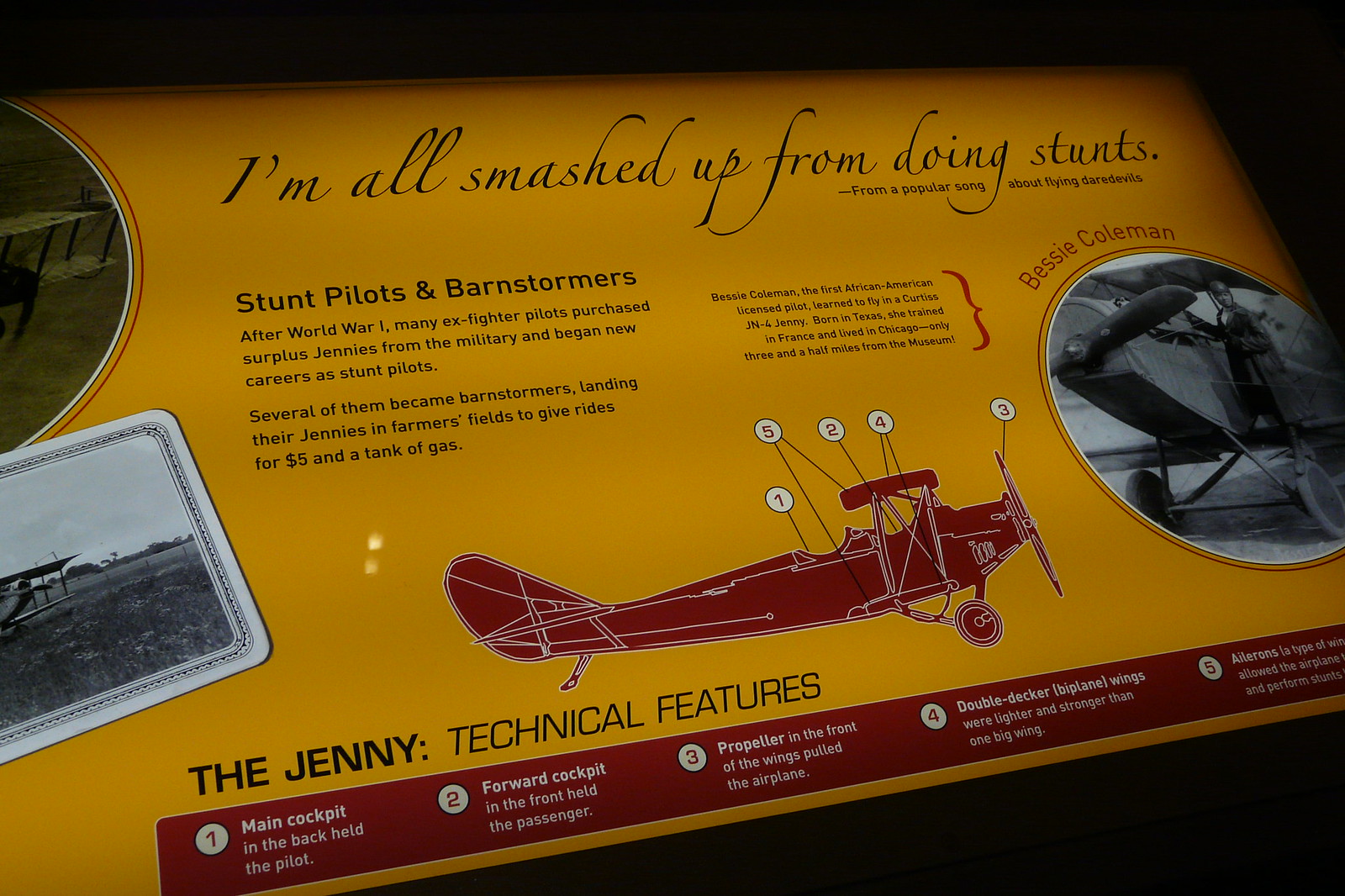The plaque, likely displayed in a museum, features a detailed and illustrative presentation of the Jenny aircraft, a historically significant plane. The plaque has a mustard yellow or orange background and is adorned with black text. At the top, a quote from a popular song about flying daredevils says, "I'm all smashed up from doing stunts." Below, the text "Stunt Pilots and Barnstormers" introduces an explanation about post-World War I pilots who bought surplus Jennys, becoming stunt performers and barnstormers, often landing in fields to give rides for $5 and a tank of gas.

On the right side, a circle encompassing a historic photograph shows a woman, identified as Bessie Coleman, standing beside a Jenny plane. Adjacent to this image, a red-colored diagram of the Jenny aircraft is labeled with numbers indicating various technical features. Specific annotations mention the main cockpit in the back for the pilot, the forward cockpit in the front for the passenger, and the propeller situated in front of the wings.

Further illustrating the aircraft, a partial black-and-white image of the Jenny is displayed on the left side of the plaque. The text "The Jenny Technical Features" and corresponding labels provide additional technical details about the aircraft, enhancing the educational value of this visually captivating exhibit.